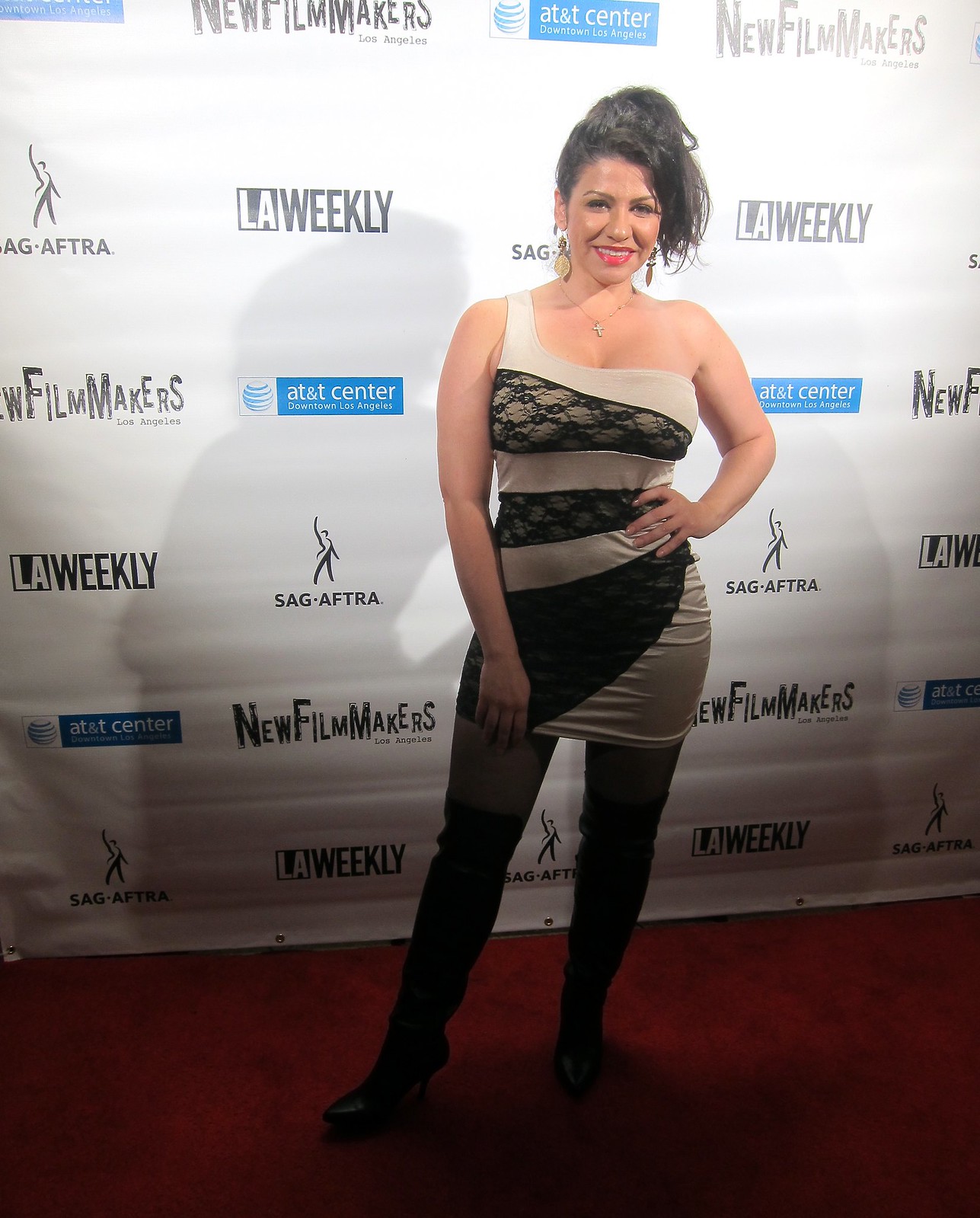The image features a woman with long black hair swept to the right, wearing a tan and black dress. The dress has a distinctive design with three black stripes over her chest, waist, and hips, with the chest and waist stripes made of lace overlay. She has a thin tan strap over her left shoulder from the viewer's perspective. The woman accessorizes with chandelier earrings, a cross pendant necklace, and black boots that reach up to her mid-thighs. She is smiling at the camera with pink lipstick on and has her right hand on her hip. The backdrop behind her is filled with logos from various organizations, including LA Weekly, SAG-AFTRA, and New Filmmakers, indicating she is at an event possibly related to the entertainment industry. The carpet she stands on is white, adding to the red carpet ambiance.